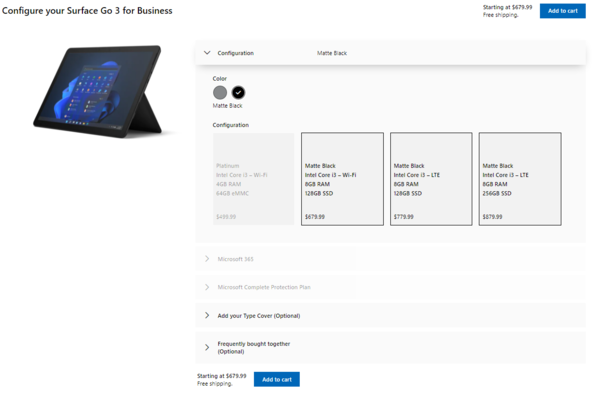The image showcases a website for configuring a Surface Go 3 for business. 

In the top left corner, the headline reads, "Configure Your Surface Go 3 for Business," accompanied by an image of the tablet placed on a stand at an angle. The tablet is powered on, displaying blue graphics and an open application or window in the center of the screen.

The top right corner of the webpage indicates the starting price of $679.99 with the promise of free shipping. There’s a prominent blue button labeled "Add to Cart."

Beneath this, a section titled "Configuration" presents a drop-down arrow. Next to this, the text "Matte Black" is displayed, with two color options indicated below: "Gray" and "Black" (with the black circle checked and labeled "Matte Black").

Further down, another "Configuration" section features four boxes: one grayed-out "Platinum" option and three "Matte Black" options. These configurations include:
- Intel Core i5 Wi-Fi, 8GB RAM, with 128GB SSD (priced at $679.99)
- Intel Core i5 LTE, 8GB RAM, with 128GB SSD (priced at $879.99)
- Intel Core i5 LTE, 8GB RAM, with 256GB SSD (priced at $879.99)

The differences between these models are explained, with the first option being Wi-Fi only, the second offering LTE capabilities with 128GB SSD, and the third providing LTE with a larger 256GB SSD.

Additionally, there is an option to add a Type Cover, which is noted as optional.